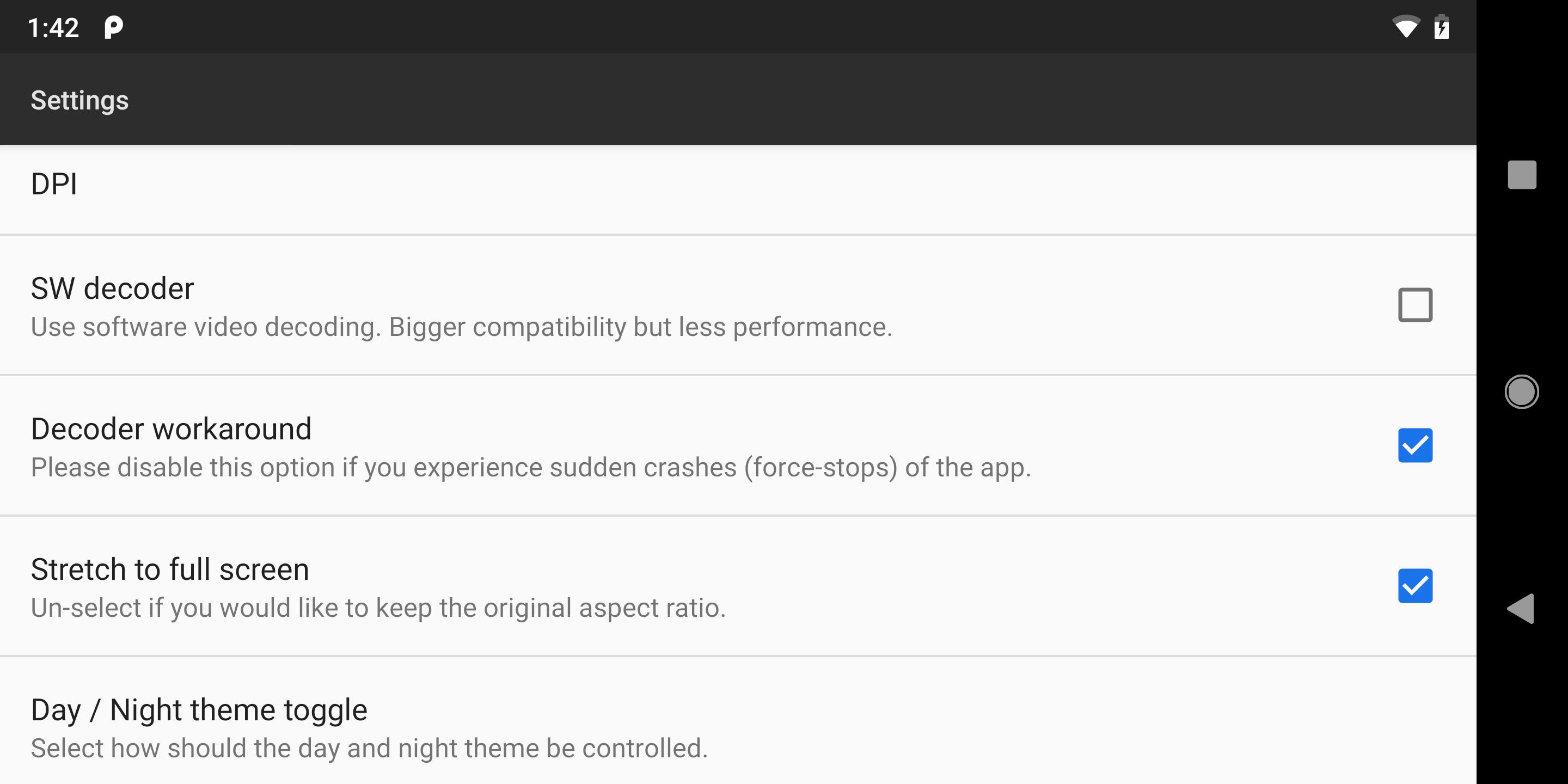A landscape-oriented screenshot captured at 1:42 PM, potentially from a smartphone or tablet, is depicted. The status bar at the top right indicates three out of four bars of Wi-Fi signal, a charging battery symbolized by a lightning bolt, and a possible hint of the Pandora app logo. 

On the right side of the screen, there are navigation icons: a square, a circle resembling a camera button, and a sideways right triangle pointing left. Below this, the screen displays a settings menu with a dark gray triangle indicating a dropdown.

The menu begins with an option labeled "DPI" followed by "SW decoder," under which the description reads, "Use software for decoding, bigger compatibility, but less performance," accompanied by an unchecked box.

Further down, "decoder workaround" is listed with a note stating, "Please disable your options if you experience sudden crashes or force stops of the app," featuring a blue-checked checkbox.

The next option, "stretch to full screen," includes the advisory, "Unselect if you would like to keep the original aspect ratio," and is currently check-marked.

Lastly, there is a "day + night theme toggle," suggesting options to select between day and night themes for better viewing preferences.